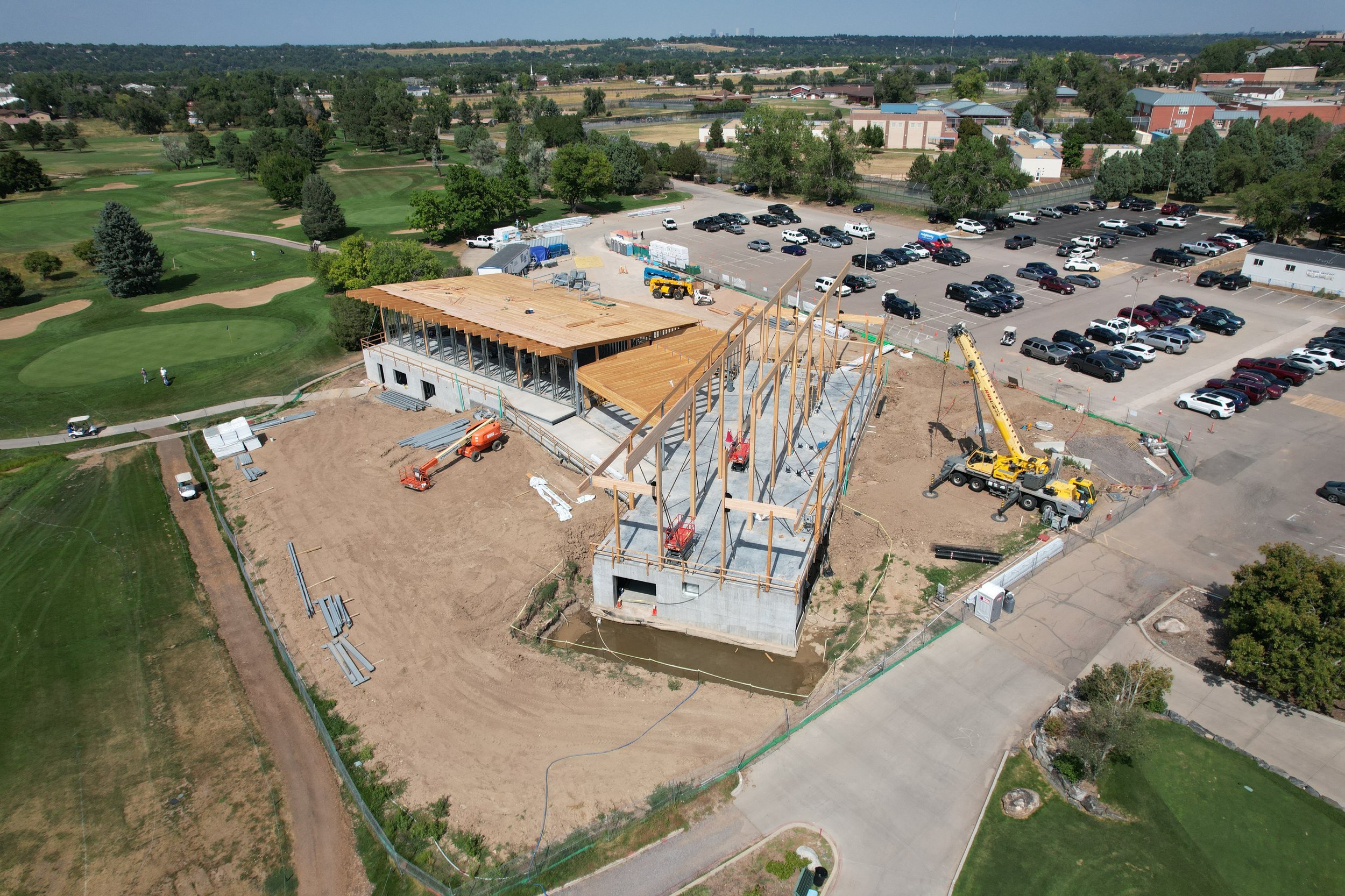This aerial photograph, likely taken by a drone, captures a detailed view of the ongoing construction of the Foothills Golf Clubhouse in Jefferson County, Colorado. The center of the image prominently features a construction zone where two buildings are being erected. A yellow crane is actively lifting wooden trusses and cross members onto a concrete base. Adjacent to the construction, on the right side, a parking area filled with numerous cars is visible, surrounded by green leafy trees and flanked by a network of roads and residential buildings. To the left of the construction site, a lush, green expanse resembling a well-maintained golf course spreads out, dotted with additional trees. The sky above is a clear blue, adding to the sharpness and clarity of the image.